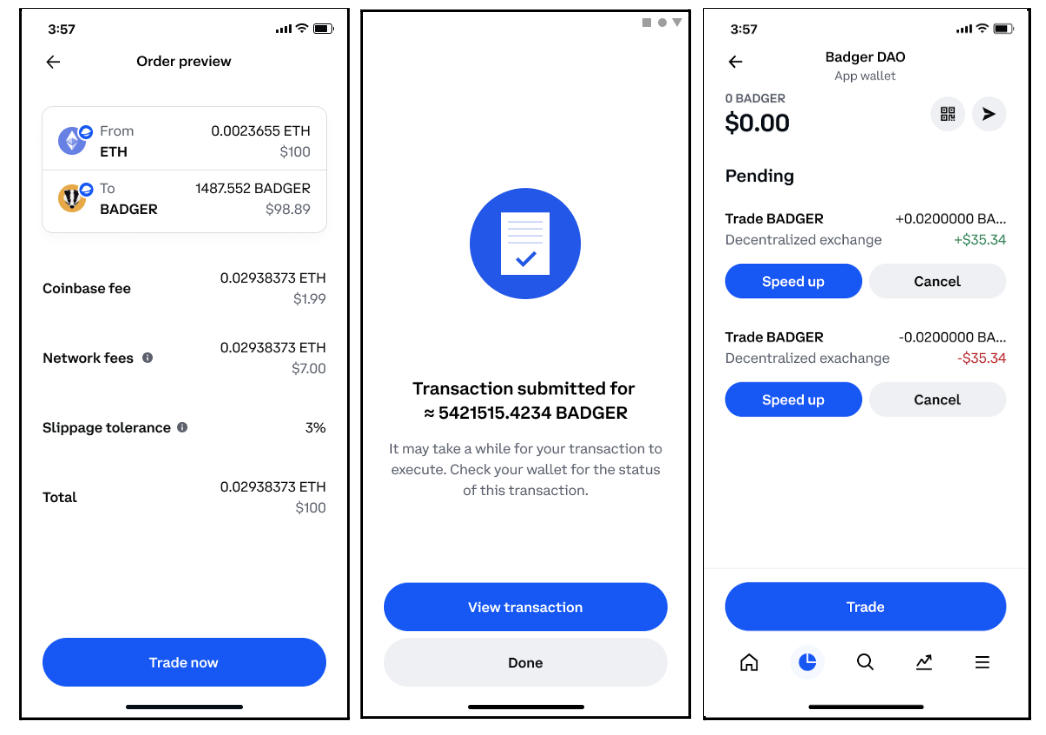Detailed Caption: 

The image consists of three consecutive screenshots captured from a smartphone at 3:57 PM, illustrating the process of a cryptocurrency transaction. 

**First Screenshot:**
The initial screen displays an "Order Preview" for a transaction converting Ethereum (ETH) to Badger. Key details shown include:
- A Coinbase fee of $1.99
- Network fees amounting to $7
- A slippage tolerance set at 3%
- A total transaction amount of $100
An option labeled "Trade Now" is prominently featured at the bottom.

**Second Screenshot:**
The subsequent screen indicates that the transaction has been submitted. There is a lengthy transaction ID provided ending with "Badger." A note advises that the transaction may take some time to execute. Below this, users are prompted to check their wallet for the transaction status, with options to "View Transaction" in blue and "Done" in gray towards the bottom.

**Third Screenshot:**
The final screen, displayed at the same timestamp of 3:57 PM, shows information from the Badger DAO app wallet:
- A balance of 0 Badger and a value of $0.00
- A pending trade of Badger with a transaction ID
Details include:
  - "Decentralized Exchange +535.34" with options to "Speed Up" or "Cancel"
  - Another line indicating "Decentralized Exchange -35.34" also with "Speed Up" or "Cancel"
At the bottom, there is an option labeled "Trade."

The entire sequence conveys an individual attempting to execute a financial transaction involving the transfer and trade of cryptocurrency through a decentralized exchange.